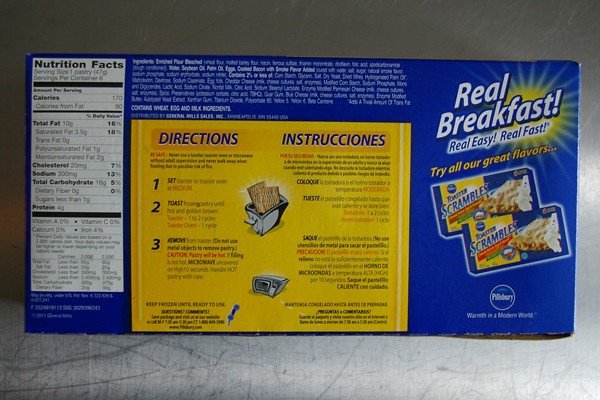The image showcases a blue-colored box taken apart to reveal three sides. The left side features a white Nutrition Facts panel detailing nutrient percentages in black text, including 170 calories per serving and 90 from fat. The central panel, the largest, contains bilingual cooking instructions—English on the left, Spanish on the right—within a prominent yellow section. This panel, which includes illustrations of a toaster ejecting the product and a microwave, likely represents the back of the box. The top strip of this panel displays ingredients. On the right, what appears to be the front of the box, a blue section promotes the product with angled white text: "Real breakfast, real easy, real fast. Try all of our great flavors," alongside images of the Toaster Scrambles and a Pillsbury logo featuring the phrase "Warmth in a modern world." Overall, the colors are predominantly blue, yellow, white, and accents of red and black text.